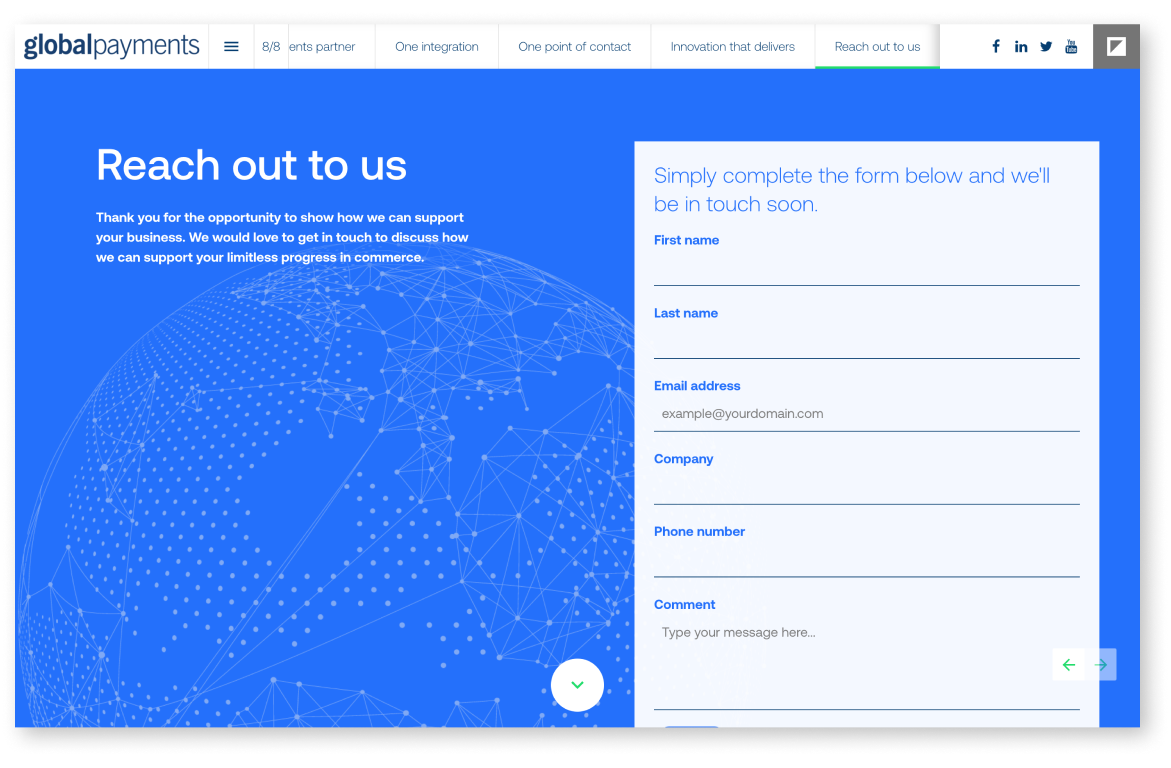This image is a detailed screenshot of a website for the company "GlobalPayments." The top border and the navigational menu are white, clearly displaying the company name in all lowercase letters. "Global" is styled in a bold, dark blue font, while "payments" is in a lighter font.

The top menu features several items: "ENTS Partners," "One Integration," "One Port," "Point of Contact," "Innovation that Delivers," and "Reach Out to Us." 

In terms of the webpage background, it is a striking shade of turquoise blue. On the left side, in white font, we see the text "Reach Out to Us." Below that, the text reads, "Thank you for the opportunity to show how we can support your business. We would love to get in touch to discuss how we can support your limitless progress in commerce."

On the right side of the screen, there is a white rectangular contact form. In blue font, the form prompts users with, "Simply complete the form below and we'll be in touch soon." The form includes fields for the user's first name, last name, email address, company, phone number, and a comment section for additional information.